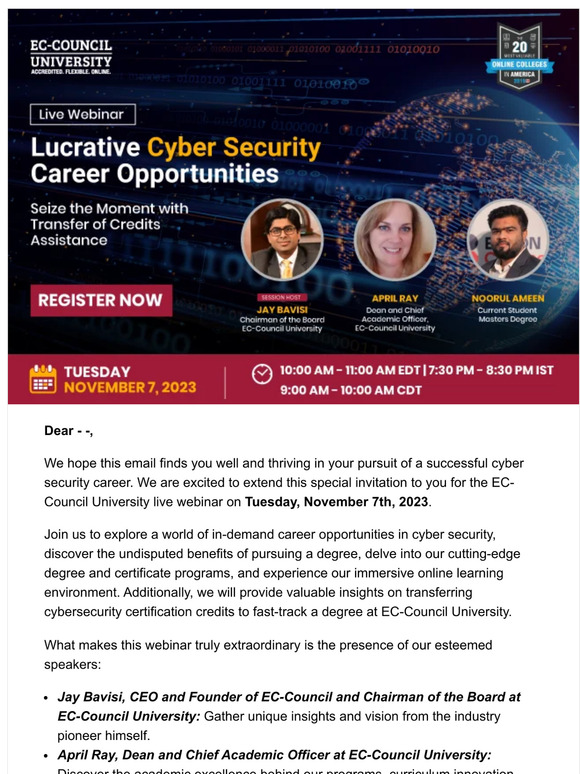The image features a grayscale, digital-themed background with a representation of the planet Earth, constructed using small, luminous dots to delineate its continents. In the upper left corner, there is text in white, which reads "EC Council University Accredited" along with additional details that are too small to discern clearly.

Prominently displayed below this text is a large header announcing a "Live Webinar" focused on "Lucrative Cybersecurity Career Opportunities." The header also includes a subtext: "Seize the moment with transfer of credits assistance."

To the bottom right of the header is a prominently placed maroon, or burgundy, call-to-action button that says "Register Now."

The lower part of the image features three circular headshots: a man on the left, a woman in the middle, and another man on the right, all set against the same burgundy border.

Centered at the very bottom is the event information within a burgundy band. It details the webinar schedule as follows: "Tuesday, November 7th, 2023, 10 a.m. to 11 a.m. EST, 7.30 p.m. to 8.30 p.m. IST, 9 a.m. to 10 a.m. CDT."

The text also includes a personalized greeting: "Dear [Name], we hope this email finds you well and thriving in your pursuit of a successful cybersecurity career. We are excited to send this special invitation to you for the EC Council University live webinar on Tuesday, November 7th, 2023."